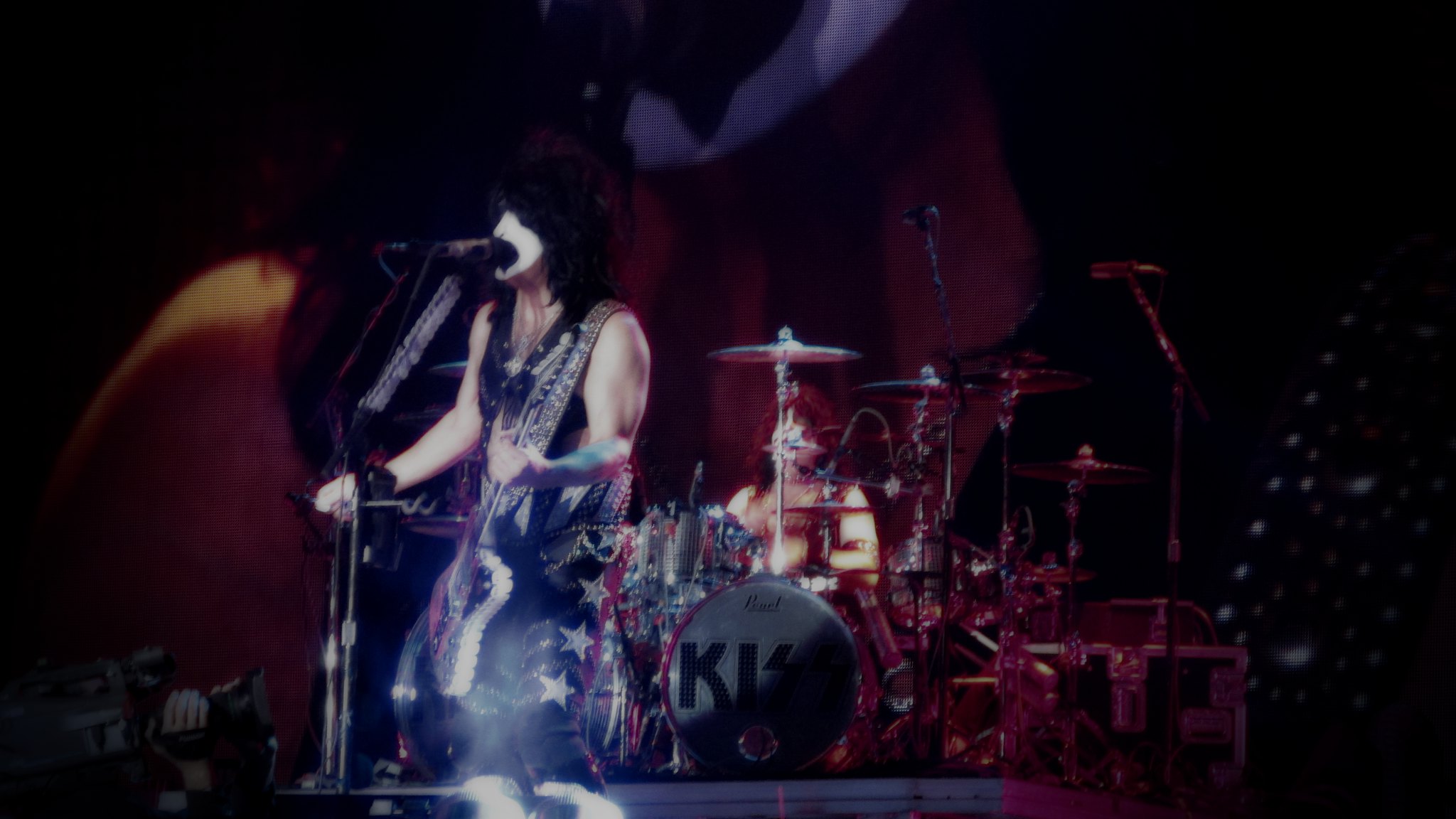This is a detailed photograph capturing a live performance by the rock band KISS, on a dark stage with subtle red lighting. Centered in the background is the drummer, partially obscured by an extensive drum kit featuring the KISS logo prominently painted on the large central drum. The drum set includes multiple cymbals and bears the Pearl logo.

In the foreground to the left, Paul Stanley is seen mid-performance, singing into a microphone while playing a white guitar with a black fretboard. He is adorned in the iconic white face makeup with black detailing, wearing a long black wig, and an elaborate costume comprised of a black leather vest and matching pants, both embellished with bedazzled stars and chains. The guitar strap is also black leather, studded with bedazzles. 

A noticeable feature to the left side of the image is a large, dark orange object, whose nature remains unclear. Additionally, a person in the lower left corner holds a large production camera, suggesting the event is being professionally filmed. The overall scene is one of dynamic energy and rock theatrics, characteristic of a classic KISS concert.